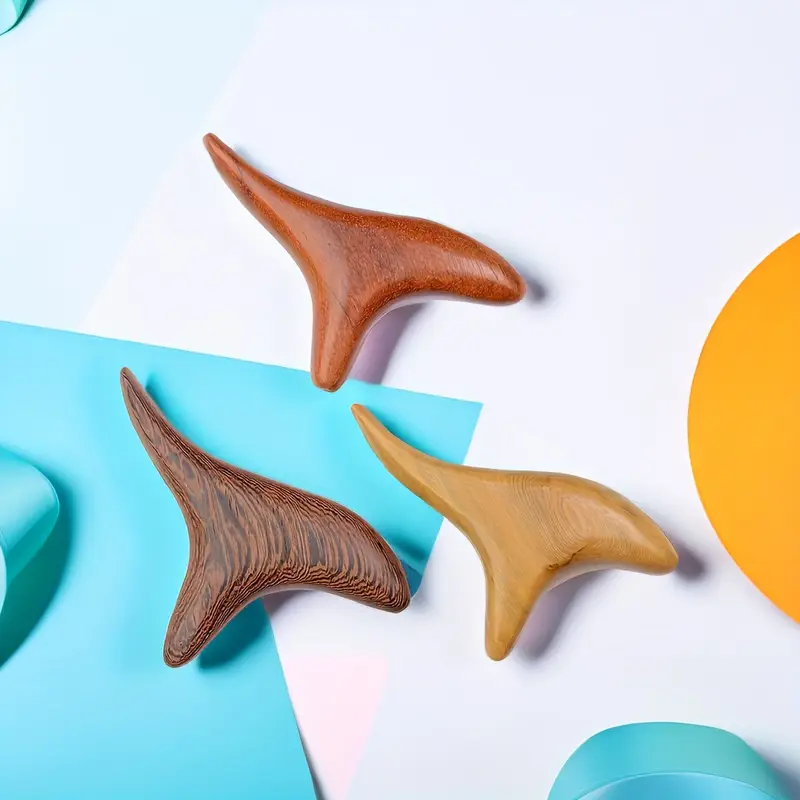The photograph captures a minimalist and abstract arrangement on a white background accented with colorful elements and uniquely shaped wooden pieces. On the far right, the edge of a yellow semicircle enters the frame, while the bottom right showcases a teal or blue semicircle ribbon-like shape. The upper left corner features a small circular blue figure, and the bottom left displays a piece of teal or light blue paper extending almost to the center, giving a layered effect to the background. Central to the composition are three distinct wooden pieces arranged in a peculiar, almost fish-like or T-shaped design with flowing curves and loops. The top piece has a reddish stain, the bottom right is a blonde pine type wood, and the bottom left is dark brown with black striping, all highly polished and artistically crafted.